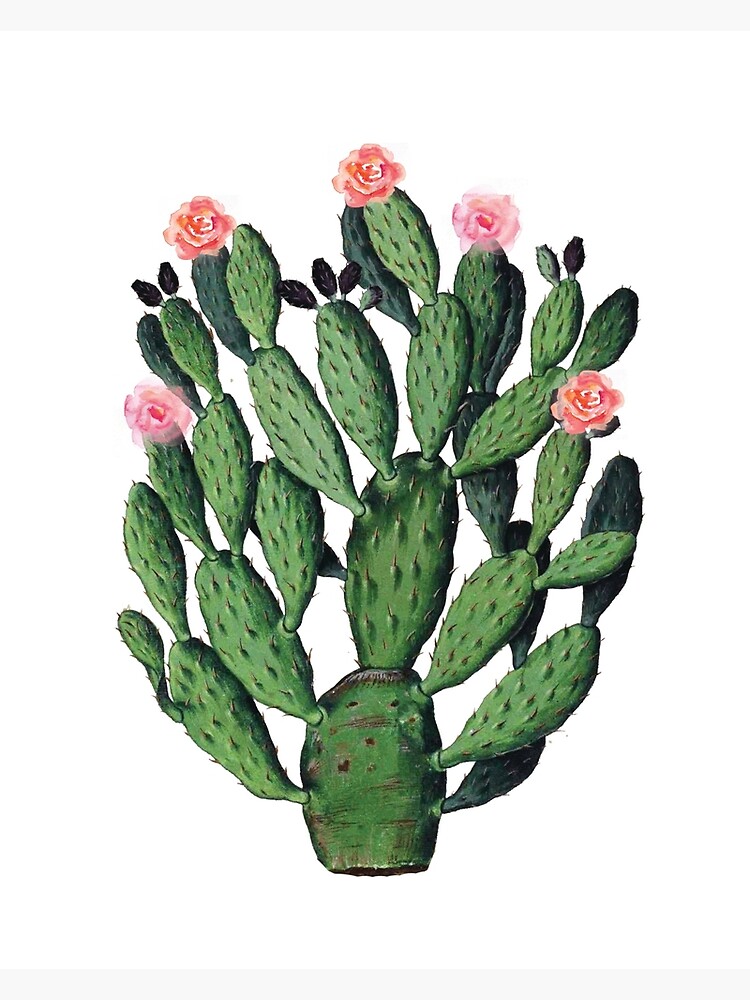This detailed painting depicts a prickly pear cactus set against a simple white background, highlighted by very faint grey rectangles at the top and bottom. The cactus starts near the bottom quarter of the frame and displays a rich palette of dark greens with various shades and brown speckles. The main body of the cactus consists of numerous lobes culminating in two prominent segments. The top segment, similar in appearance but adorned with brown spikes instead of speckles, further branches into smaller pale green lobes. Each of these has additional brown spikes and smaller dark brown lobes clustered in pairs of two or three. Watercolor brushed pink flowers, totaling five, bloom from the tips of the farthest lobes, arranged in a graceful arc. The image is well-shaded with a realistic style, capturing the cactus in full bloom with a dense array of segments and thorns, offering a clear and vibrant depiction of a healthy plant.